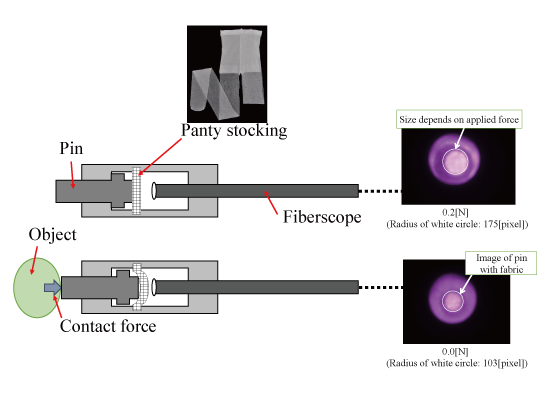This detailed technical rendering displays an experimental setup involving pantyhose. At the top, a small black box labeled "Panty Stocking" features a white pair of pantyhose with a red arrow pointing downward. The arrow leads to a gray diagram with the word "PIN," next to which the word "Fiberscope" is labeled. This connects to another black box that states, "Size Depends on Applied Force." 

On the left side of the diagram, a green circle labeled "Object" has an arrow pointing down with the term "Contact Force" beside it. The Fiberscope connects this to another black box showing "Image of Pin with Fabric," highlighting a purple circle with text below it that reads "Radius of white circle, 103 pixel."

Further examination in the bottom right reveals a secondary black square, again containing a purple circle, this one annotated "Size Depends on Applied Force." Beneath this entry, it reads, "Radius of white circle, 175 pixel." This entire setup demonstrates the relationship between applied force and the resulting image size captured when examining the fabric of pantyhose under a fiberscope.